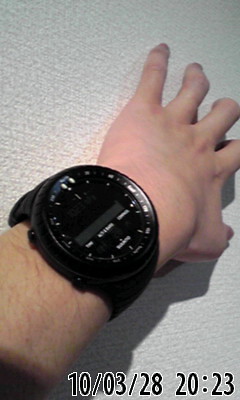In this detailed photograph, a person's left hand, with fair skin and light arm hair, prominently displays a large black wristwatch. The watch features a wide black dial and a matching band, which appears oversized for the wrist. The wristwatch face, occupying almost the entire width of the wrist, shows the current date, 10/03/28, in black characters. The time displayed is 20:23, also in black, with a colon separating the hours and minutes. White numerals and letters contrast sharply against the black background of the watch's dial. The background of the image is a white surface accented with beige striations. A noticeable black shadow falls across the lower left corner of the photograph, adding depth to the setting. The hand itself is slightly blurry, suggesting a casual, unposed snapshot, possibly taken of a younger individual or an adolescent. The primary focus of the image is undoubtedly the wristwatch, which seems to be emphasized by the added date and time details, likely indicating an international context such as March 28th, 2010.